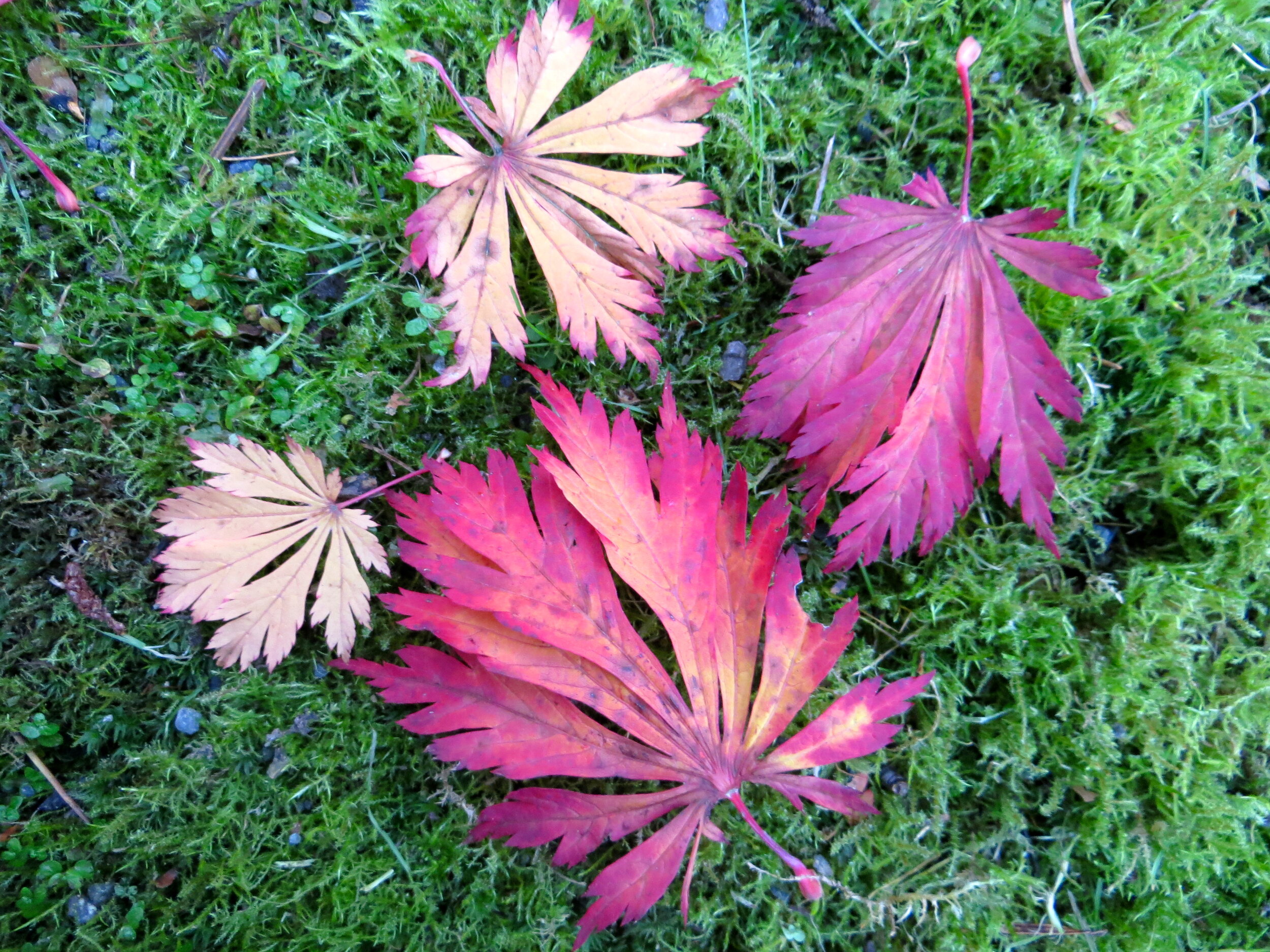This detailed photograph captures an outdoor scene with a vibrant base of green grass interspersed with clovers and small blue flowers, possibly indicative of a lush, natural setting. Laid out in an artistic arrangement on the grass are four distinctly beautiful leaves, resembling those of a Japanese maple. These leaves showcase a striking palette of colors: the largest leaf at the bottom boasts a mesmerizing blend of pink-purple and yellow hues. To the top right, an upside-down leaf exhibits darker, more pronounced purple tones alongside similar yellow accents. The smaller leaves to the left and at the top present lighter shades, with one appearing whitish tan and the other adorned with subtle purple tipping. Together, the leaves, with their intricately cut shapes and dynamic coloration, create a visually captivating tableau against the verdant ground cover.